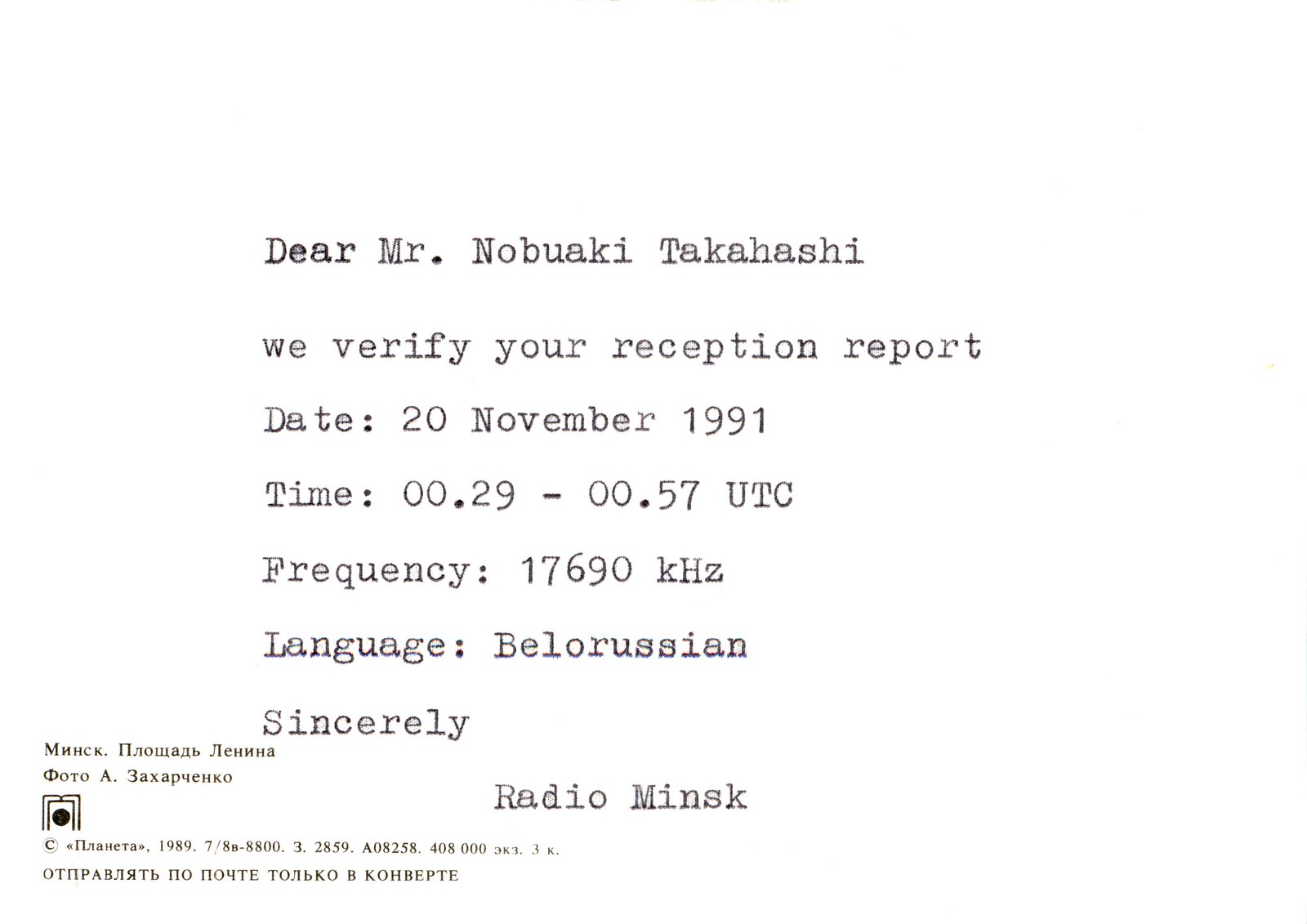The image presents a white graphic resembling a transmission verification or confirmation document. The text appears to be typed on a typewriter, with some characters showing ink bleeding into the paper. It reads: "Dear Mr. Nobuaki Takahashi, we verify your reception report, date: 20 November 1991, time: 00.29-00.57, UTC, frequency: 17690 kHz, language: Belarussian, sincerely, Radio Minsk." In the bottom left corner, there are four lines of small text, including a logo in the middle. The text is written in a language that appears to be Russian.